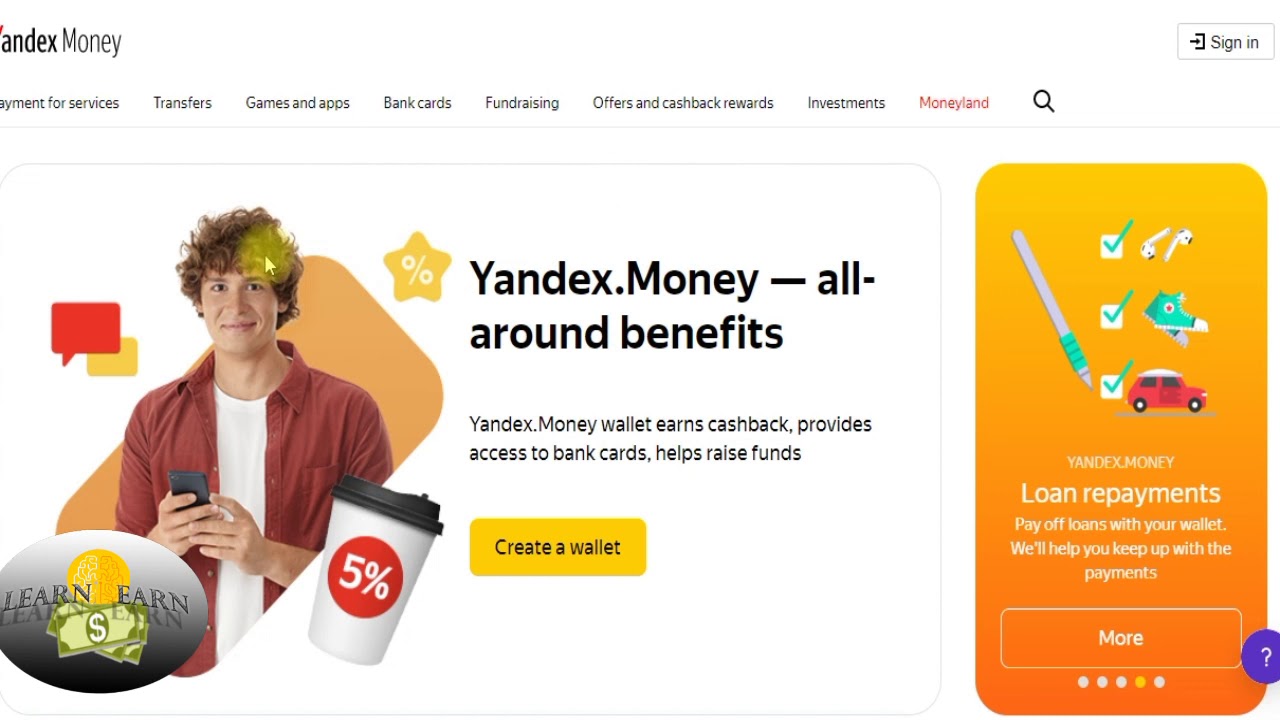This image features a screenshot of the Yandex Money website. The upper left-hand corner prominently displays the "Yandex Money" logo, though the 'Y' is partially cut off due to the image crop. The 'Y' in "Yandex" is capitalized and bold, while "money" is also capitalized but not bold.

Below the logo, there's a horizontal menu bar with options: "Payment for Services," "Transfers," "Games and Apps," "Bank Cards," "Fundraising," "Offers and Cashback Rewards," and "Investments." Further options appear to be partially visible but cut off by the image's edge.

The main section of the website features an image of a man using a cell phone, directly engaging with the camera. The man is dressed in a long-sleeve red shirt. Accompanying the image is a floating coffee cup icon with a "5%" label, likely indicating a discount or reward. Adjacent to this is a red text bubble, adding context or additional information related to the image and the coffee cup. 

This detailed scene captures a blend of digital and lifestyle elements designed to enhance the user experience on the Yandex Money platform.